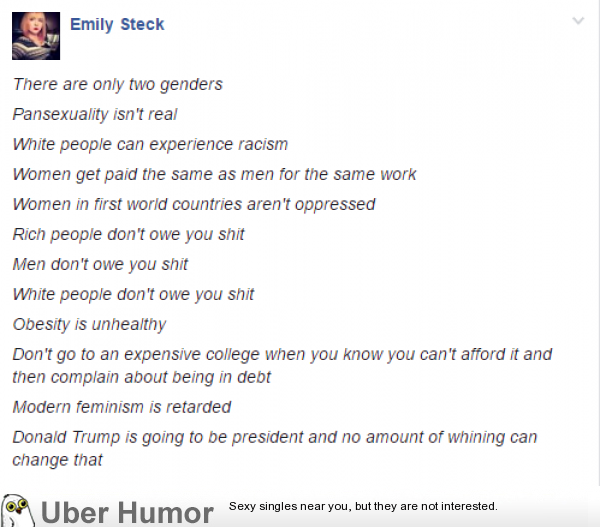In this image, we see Emily Steck dressed in a casual outfit, standing against a plain white background. The text overlay, written in italics, seems to be a provocative and controversial social media post, possibly from Facebook. The message includes multiple statements addressing various societal issues:

"There are only two genders. Pansexuality isn't real. White people can experience racism. Women get paid the same as men for the same work. Women in first-world countries are not oppressed. Rich people don't owe you anything. Men don't owe you anything. White people don't owe you anything. Obesity is unhealthy. Don't go to an expensive college if you know you can't afford it and then complain about debt. Modern feminism is flawed. Donald Trump is going to prison."

A humorous addition follows, with a bird illustration and text alluding to "sexy singles near you," suggesting a satirical tone. The background of the post is white, emphasizing the bold claims made in the text, which are meant to provoke discussion or highlight particular viewpoints.